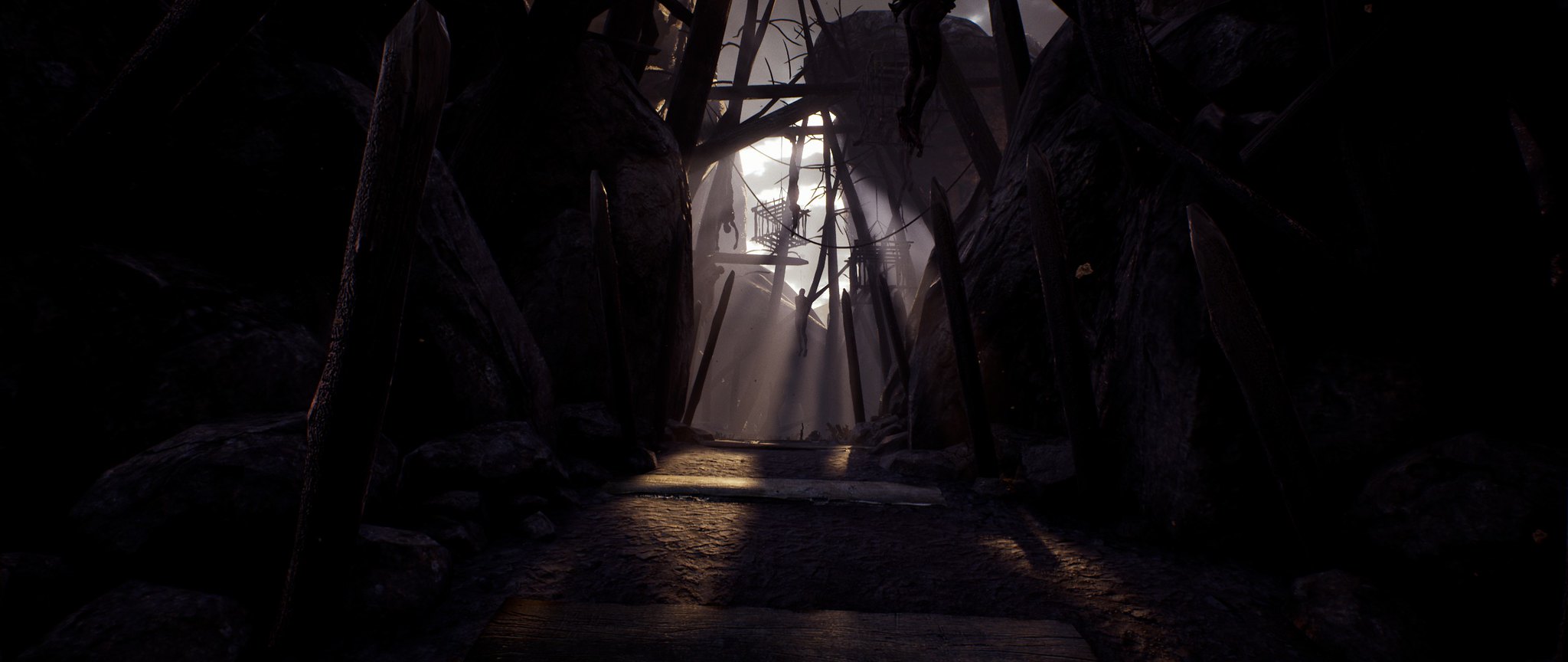A dark, atmospheric scene from a computer game, possibly set within a cave or cave-like structure. Sunlight penetrates through an opening, illuminating scattered wooden debris on the ground and partially revealing wooden structures outside the cave. In the distant background, a patch of blue sky with a hint of a white cloud is visible. A square cage is prominently placed within the frame. The surrounding areas remain shrouded in shadow, creating a mysterious and foreboding ambiance.